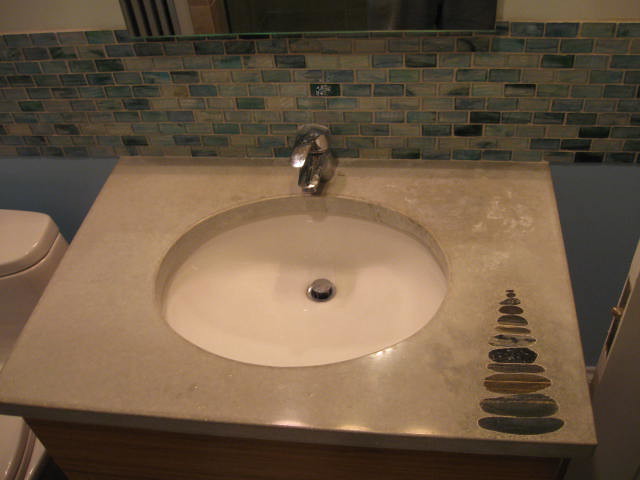This image features a bathroom sink as its central focus. The sink has a circular basin with a whitish hue and is set into a stone countertop. The countertop exhibits a unique ribbed pattern on the right-hand side, starting small and progressively enlarging. Directly above the sink, the wall is adorned with small, intricately placed tiles in shades of teal and blue. A sleek silver faucet complements the elegant setup of the sink area.

On the left side of the photograph, part of a white toilet is visible, though it's largely obscured by the framing of the image. To the right, there's an open door that slightly intrudes into the shot, its full details obscured but with hints of a blue wall visible on either side in the background. The balanced use of color and texture creates a visually appealing and inviting atmosphere in this bathroom space.